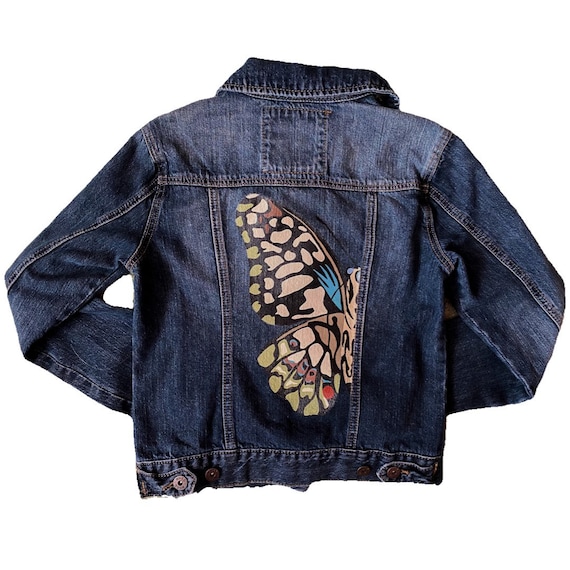The image features the back of a classic Levi’s denim jacket, positioned against a white backdrop. The jacket is a deeper, darker blue shade typical of Levi's. A central butterfly pattern dominates the back panel of the jacket, featuring intricate details of wings with colors primarily in black, beige, and red, along with some blue and turquoise highlights. The pattern includes one eye and parts of the left wings, with elements of green and flesh tones against a black background. 

The jacket itself retains traditional Levi’s features, including detailed etchings on the denim and four classic copper-toned buttons at the bottom, near a double-seamed waistline. The arms of the jacket are posed slightly bent, emphasizing the butterfly design and its placement between two vertical seams. The stitching throughout the jacket corresponds with Levi's distinguished craftsmanship.